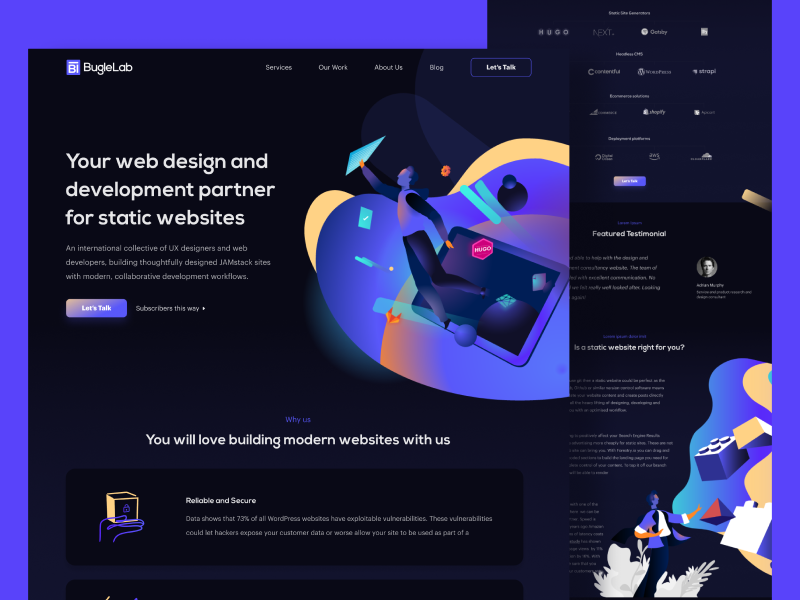In this image, a vibrant and meticulously designed webpage is displayed. The background is a striking bright purple with sheer black overlays, while the main text is depicted in clean white. The top-left corner features a logo within a purple square: a white bee encased in a horizontal and vertical border, accompanied by the text "Bugle Lab". 

To the right of the logo, along the upper margin, are navigation links in white text: "Services", "Our Work", "About Us", "Blog", and a prominently highlighted "Let's Talk" in bolded bright purple.

Dominating the central area of the webpage is a large, bold header in white: "Your Web Design and Development Partner for Static Websites". Beneath this, a descriptive subheading reads: "An International Collective of UX Designers and Web Developers Building Thoughtfully Designed JAMstack Sites with Modern Collaborative Development Workflows." Positioned below this text is a purple rectangular button with white lettering: "Let's Talk", alongside a prompt in white: "Subscribers This Way".

Adjacent to this text is a futuristic, computer-animated style illustration, rendered in smooth shades of yellow, blue, purple, orange, black, gray, and pink. The illustration features a floating tablet, various abstract shapes, gears, orbs, and a stop sign labeled "Hugo". A man, in side profile with dark pants, a light-colored shirt, and short, dark hair, is depicted reaching upwards with his right hand towards one of the floating shapes.

Below the main illustration, purple text introduces a section titled "Why Us", followed by bolded white text stating: "You Will Love Building Modern Websites With Us". Further down the page is a black rectangular section with white text detailing the benefits: "Reliable and Secure. Data shows that 73% of all WordPress websites have exploitable vulnerabilities. These vulnerabilities could let hackers expose your customer data or, worse, allow your site to be used as part of A."

In the bottom right-hand corner, another futuristic illustration in similar smooth shades of yellow, purple, blue, orange, pink, and white is visible. This scene features several floating, blocky shapes reminiscent of Lego blocks in white and blue. A man is again pictured in side profile, reaching towards the floating blocks above an irregular blue blob.